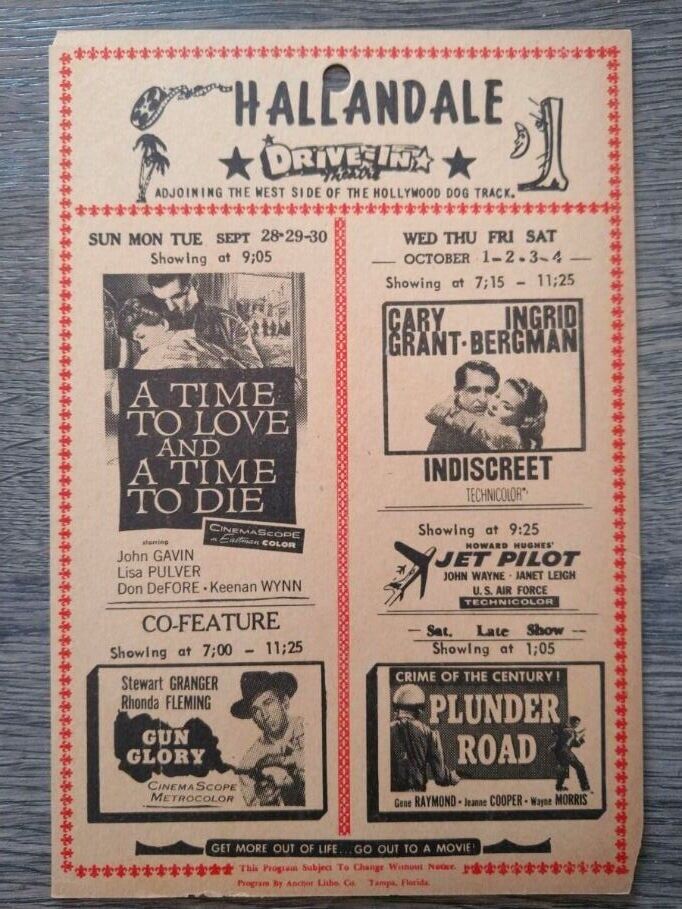This is a vintage promotional flyer for the Hallandale Drive-In Theater, likely from the 1950s or 60s, characterized by its worn white background with distinct red borders and dividing lines. The top half of the flyer prominently features the theater's logo, which reads "Hallandale Drive-In Theater," flanked by two filled-in black stars. To the right of the logo, there's an image of a moon beside a speaker set, while to the left, a film reel being pulled with part of the film visible, accompanied by a small palm tree. 

Beneath the logo, the flyer states the location "Adjoining the West Side of the Hollywood Dog Track." The flyer is divided vertically into two sections, each showcasing different movie listings. On the left side, two movies are advertised: "A Time to Love and A Time to Die," showing on September 28, 29, and 30 at 9:05 PM, which features stars John Gavin, Lilo Pulver, Don DeFore, and Keenan Wynn, depicted with an image of a man holding a woman close. Below it, the co-feature "Gun Glory" is advertised, showing from 7:00 PM to 11:25 PM, starring Stewart Granger and Rhonda Fleming. The associated image shows a man wearing a cowboy hat, shooting a revolver.

On the right side, the flyer promotes "Indiscreet" featuring Cary Grant and Ingrid Bergman, which is scheduled from October 1 to 4 at 7:15 PM to 11:25 PM, and depicted with an image of a woman hugging a man from the back. Below it, "Jet Pilot" by Howard Hughes, starring John Wayne and Janet Leigh, is slated to show at 9:25 PM, illustrated with two fighter jets. The Saturday Late Show at 1:05 AM features "Crime of the Century" and "Plunder Road," depicted with an image of a man wearing a helmet and another person skulking. The flyer concludes with the slogan "Get More Out of Life, Go Out to a Movie" and a note indicating the program’s subject to change, mentioning a company based in Tampa, Florida. The entire flyer appears to be set on a wood-paneled surface.